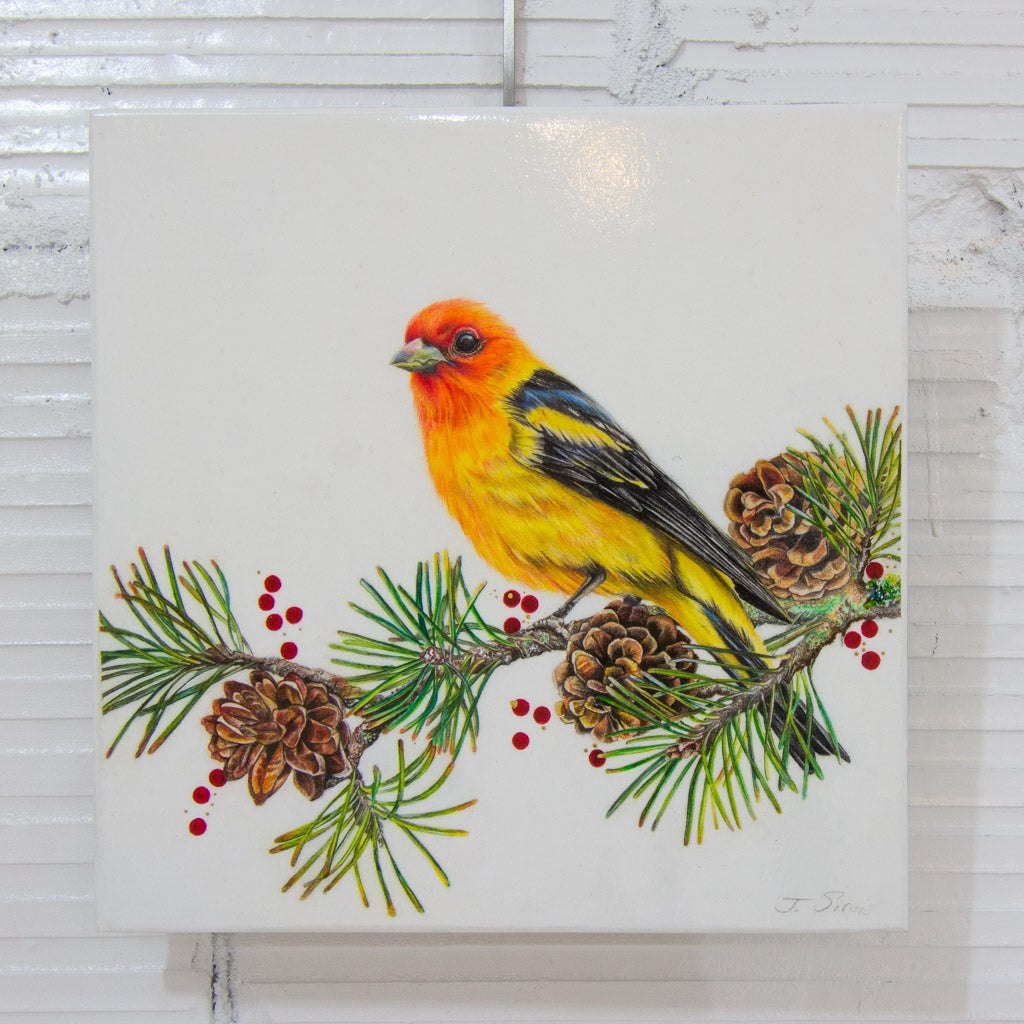The image depicts a detailed painting of a vibrant Oriole perched on a pine branch. The bird, primarily yellow with an orange to red head, sports black wings accented with yellow markings and a gray beak. The branch features three prominent pine cones, evergreen needles, and numerous small red berries scattered along it. The painting is signed in the bottom right by J. Siron, with the signature partially obscured. The artwork is presented on a glossy, reflective white canvas, suspended by a metal rod, and is set against an old, textured white concrete wall with slight ridging.